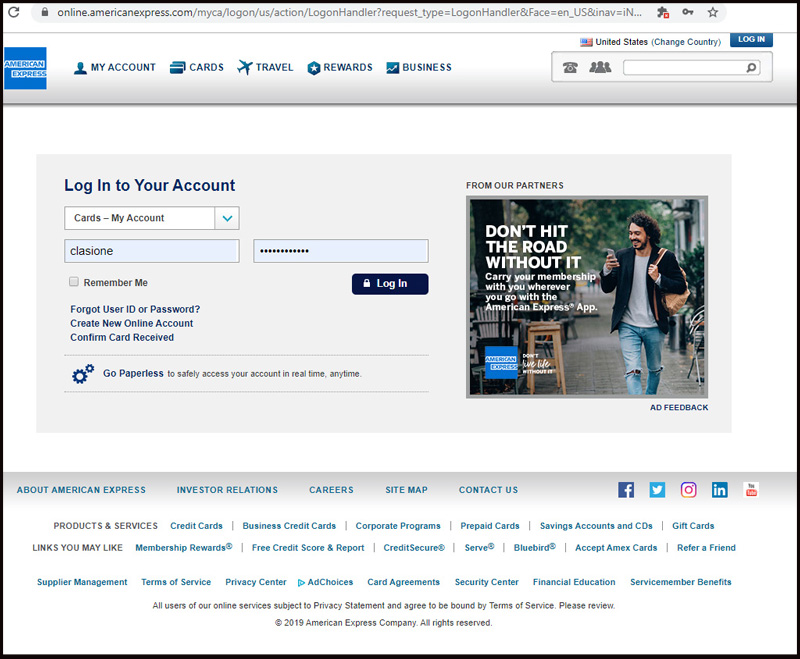**Caption:**

This image is a vintage screenshot from the American Express website, exhibiting a design style characteristic of the early 2010s, around 2010-2012. The web address at the top indicates the URL, online.americanexpress.com, with a notably long string following it. The page features a silver-gray header with the American Express logo prominently displayed on the far left, showcasing the iconic blue background with "American Express" written in blue and outlined in white.

This screenshot captures the login page, with a top menu listing options from left to right: My Account, Cards, Travel, Rewards, and Business. Central to the page is a large gray rectangle containing the login interface. The header within this section reads "Login to Your Account," with a dropdown menu labeled "Cards, My Account" for users to select their login type. Below are two input fields for entering a username and password, followed by a dark gray oblong login button with the word "Login" in white text.

Adjacent to the login section is an advertisement featuring a white male model, who has long brown hair, a beard, and a mustache. He is dressed in a blue shirt, ripped and faded cut-off jeans, and a black jacket, holding a smartphone in his hand. The ad's headline, presented in white font, reads "Don't Hit the Road Without It. Carry your membership with you wherever you go with the American Express app." The familiar blue American Express logo is displayed again in the lower left-hand corner of the ad, reinforcing the brand identity.